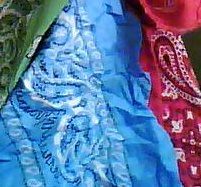The image is a very close-up, square photograph of three bandanas layered on top of one another, highlighting every wrinkle in the fabric. In the top left corner, there is a partial view of a dark green bandana adorned with light green and white paisley patterns. The middle bandana, the largest, is a shade of light blue with intricate white and dark blue designs. On the right, there is a partial view of a classic red bandana featuring prominent white and black paisley prints. In the upper right corner, a reddish-pink sleeve intrudes slightly into the frame, adding an unintended splash of color. The background of the image has hints of black, contrasting with the vibrant colors of the bandanas.